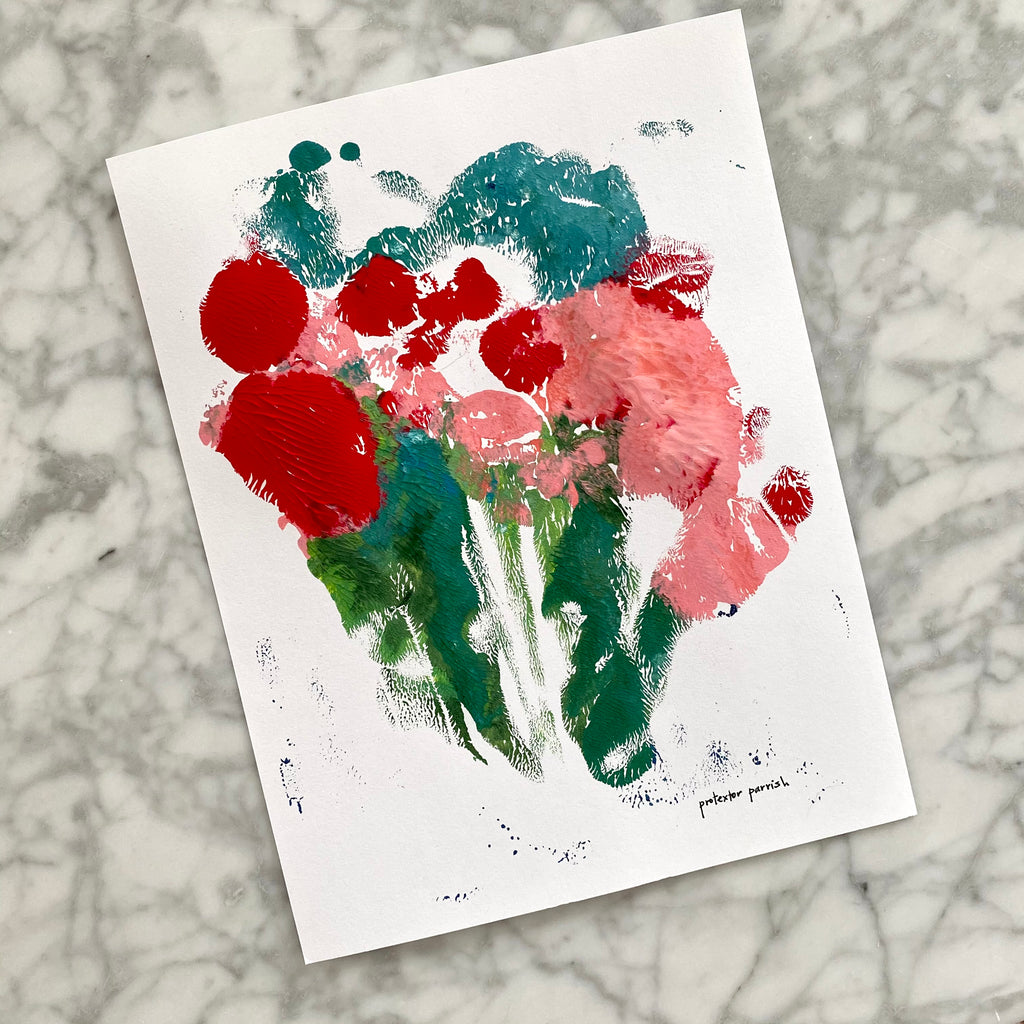This photograph features an abstract painting on a piece of thick, cardstock-like paper, set upon a white and gray marble surface and tilted slightly to the left. The vibrant artwork, potentially created with oil-based paints, showcases a rich texture and brush strokes that are clearly visible. The painting is open to interpretation, with color splashes of red, pink, green, teal, aqua, and white blending in various patterns. Notably, the left side features two circular shapes in red, while the right side displays a beaver-shaped pink form. Green foliage extends downward from the red circles, and a thin, green spiral emerges from the pink shape. Above the pink form is an aqua-greenish color resembling an elephant’s head, accompanied by similar splashes above the top red circle. The painting, which may evoke floral imagery with green stem-like structures and colorful flower representations, is signed "Protector Parish" at the bottom. The marble countertop beneath suggests a domestic setting, possibly a kitchen.